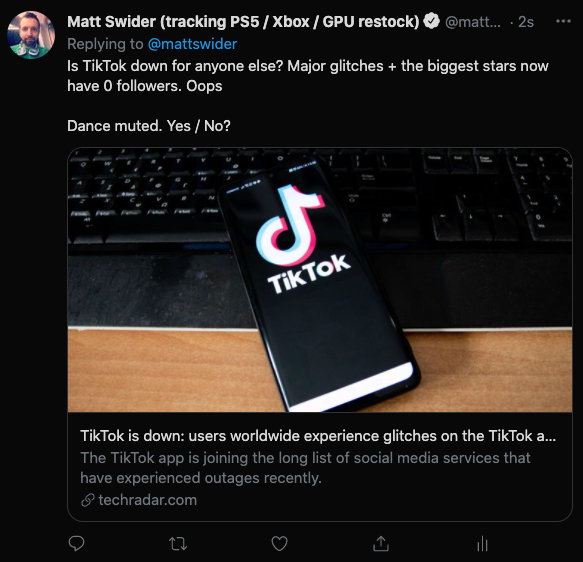**Descriptive Caption:**

"A screenshot of a Twitter post by Matt Sweider, whose profile mentions that he tracks restocks for PS5, Xbox, and GPU. The tweet was posted just two seconds ago and is a reply to his own account, @MattSweider. In the tweet, Matt inquires if TikTok is down for others, citing major glitches and noting that prominent users have suddenly lost all their followers. The tweet humorously ends with 'Dance muted yes/no' and includes a link to a TechRadar article titled 'TikTok is down: Users worldwide experience glitches on the TikTok app.' The remaining text of the article snippet mentions that TikTok is joining a growing list of social media platforms experiencing outages recently."